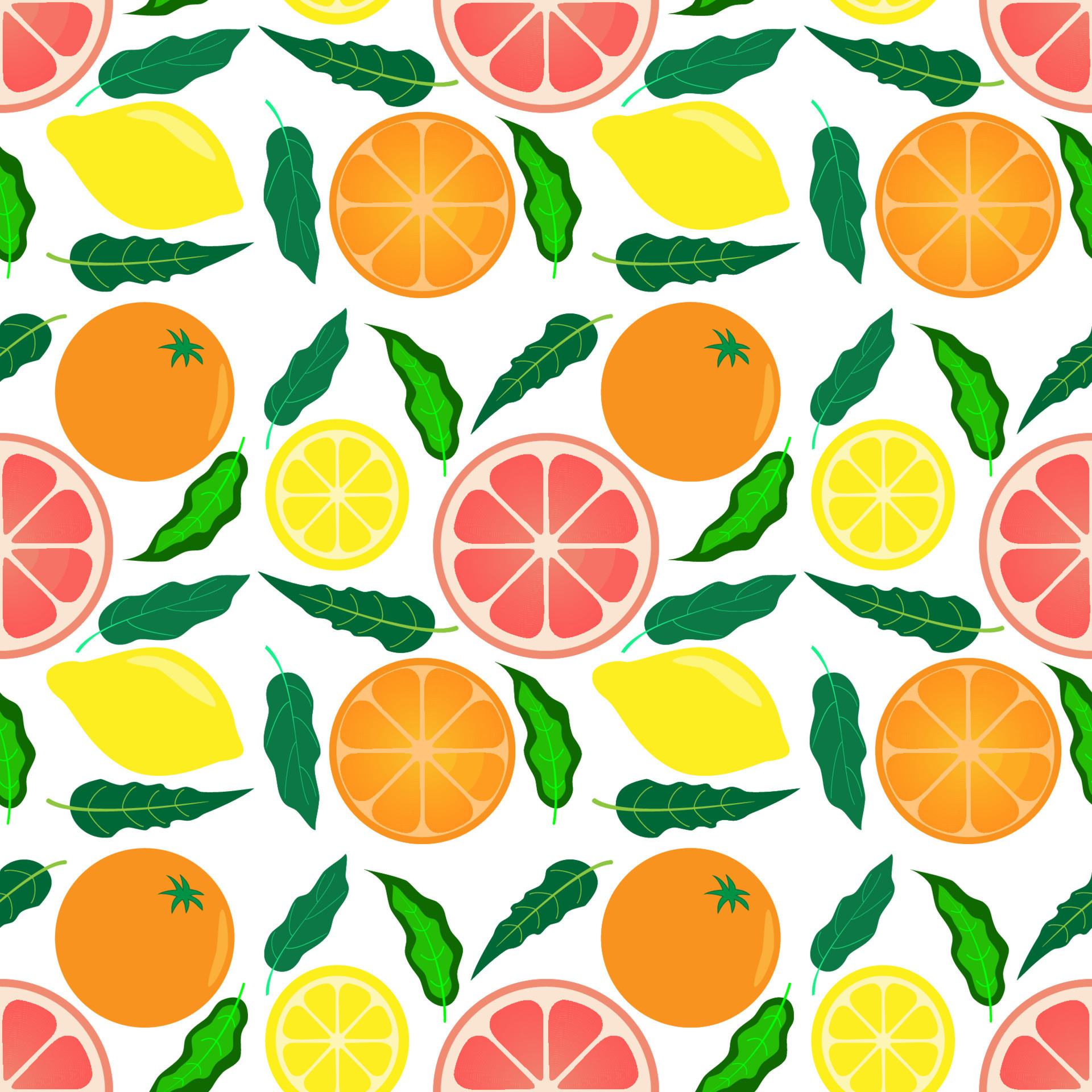A vibrant arrangement of citrus fruits is beautifully displayed on a pristine white cloth. A sliced orange, showcasing its juicy segments, sits alongside a whole orange adorned with a small green stem. Dotted between these are lush green leaves, adding a fresh, lively touch. A slice of bright yellow lemon contrasts against the vivid colors, while a generous slice of pink grapefruit adds a splash of rosy hue. Scattered throughout are additional whole lemons, whole oranges, and more pink grapefruit slices, each interspersed with more green leaves. The leaves have jagged edges and sharp points, enhancing the natural, organic feel of the composition. The combination of bright orange, cheerful yellow, and soft pink fruits against the clean white background, all accented by the striking green foliage, creates a stunning and refreshing visual feast.